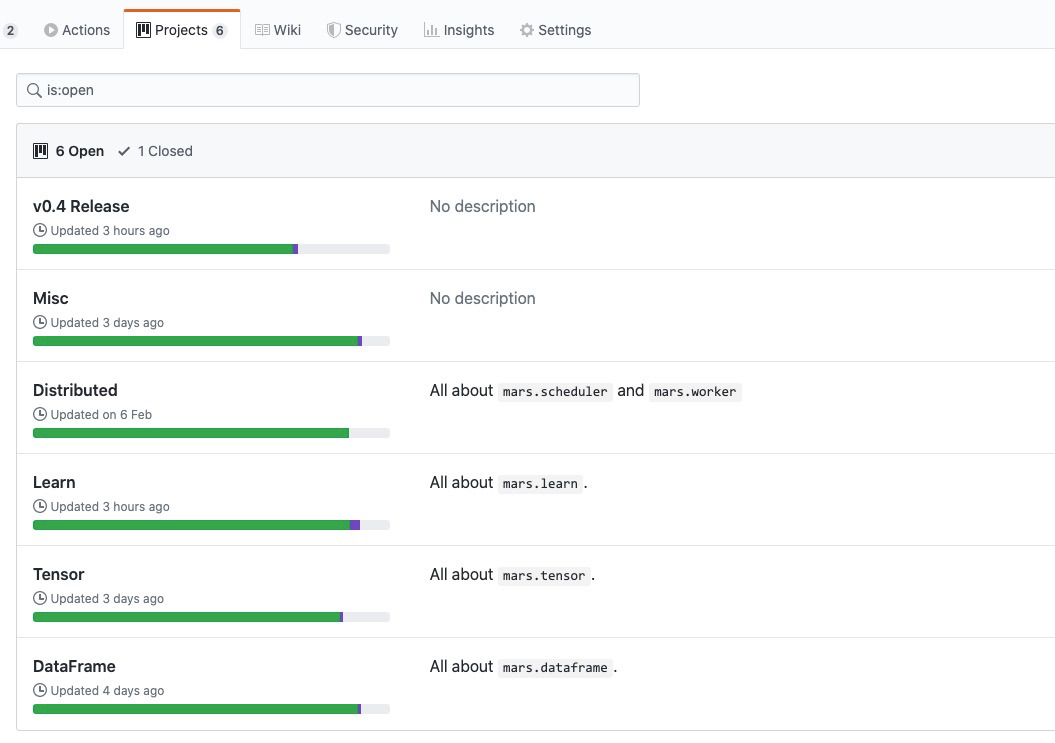The image is a screenshot of a web application's interface, reminiscent of a desktop view, where the width is significantly greater than the height. The interface predominantly features a crisp white background contrasted by black text. Green progress bars span from left to right, visually representing the progress or completion status of various tasks.

At the top of the interface, there's a header populated with several clickable tabs designed for navigation. These tabs are labeled: Actions, Projects, Wiki, Security, Insights, and Settings. The Projects tab is actively selected, highlighted by a small number six adjacent to it, indicating the presence of six projects.

Below the header, a detailed table lists the various projects and their statuses. It specifies that there are six open projects and one closed project. The first project listed is titled "Version 0.4 Release," albeit without a description. It displays a green progress bar extending about four-fifths of the way across the screen, denoting substantial completion, and notes that it was updated three hours ago.

Further down, other projects named Miscellaneous, Distributed, Learn, Tensor, and DataFrame are listed, each presumably accompanied by their respective progress indicators and last updated timestamps, providing a comprehensive overview of the current project statuses within the application.